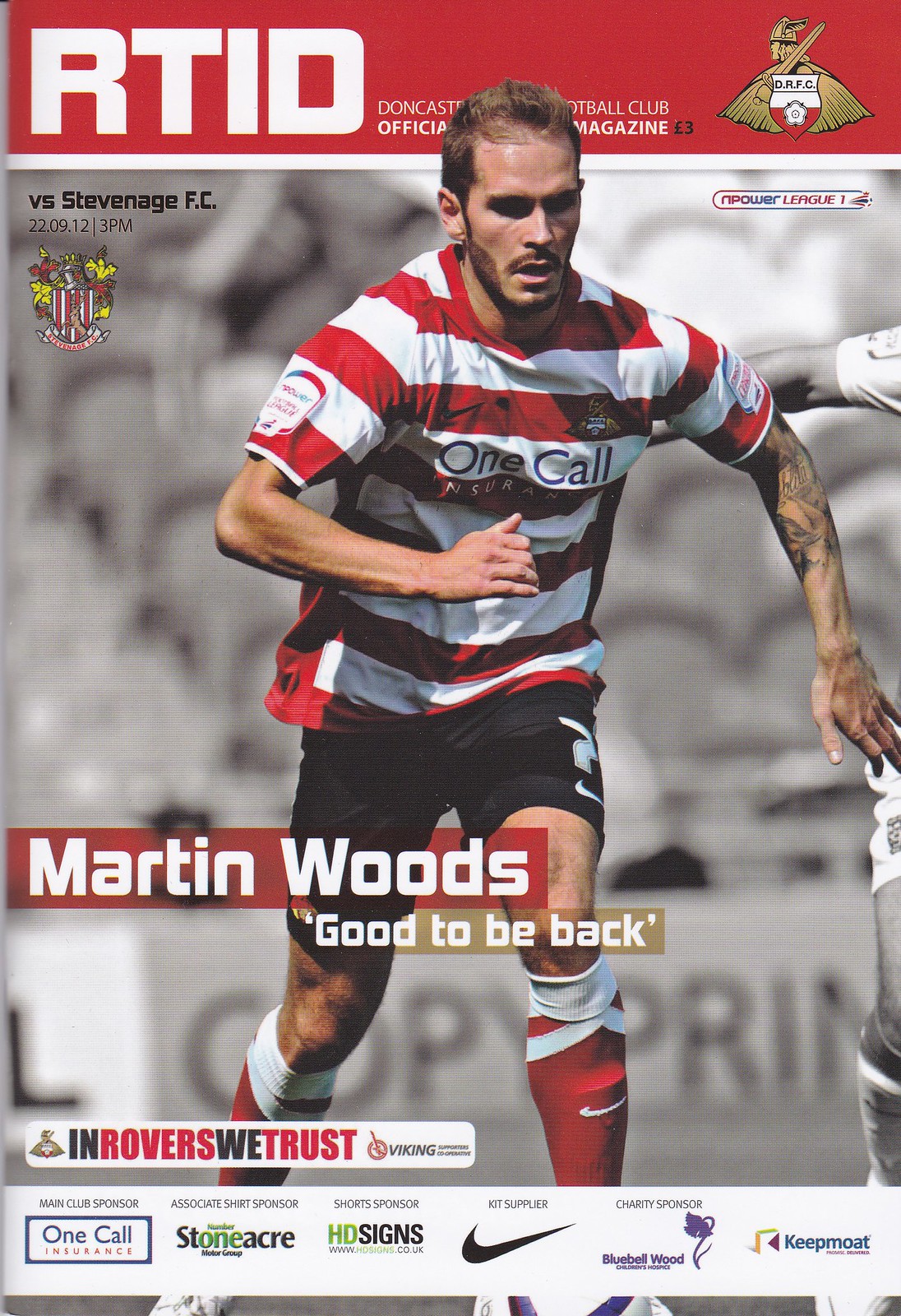The cover of the RTID Doncaster Football Club official magazine features a dynamic image of soccer player Martin Woods. Central in the portrait-oriented layout, Martin Woods is captured in motion, running on a field while wearing a red and white horizontally striped shirt, black shorts, and knee-high red socks. Notably, he has a tattoo on one arm and brown hair. The backdrop of the image is a striking black and white, making Woods stand out prominently.

At the top of the magazine cover is a bold red bar with large white text proclaiming "RTID" and a gold, red, and white logo featuring a Viking with a sword on his shoulder and a shield marked "DRFC." Below this, a red bar with white text overlaid at Woods' knees reads "Martin Woods" and a gold bar underneath it declares "Good to be back."

Towards the bottom of the cover, a white banner filled with colorful sponsor logos includes One Call Insurance, Stoneacre, HD Designs, Nike's iconic swoosh, Bluebell Wood, and Keepmoat. The slogan "In Rover We Trust" is also featured prominently, conveying the pride and unity of the club and its supporters.